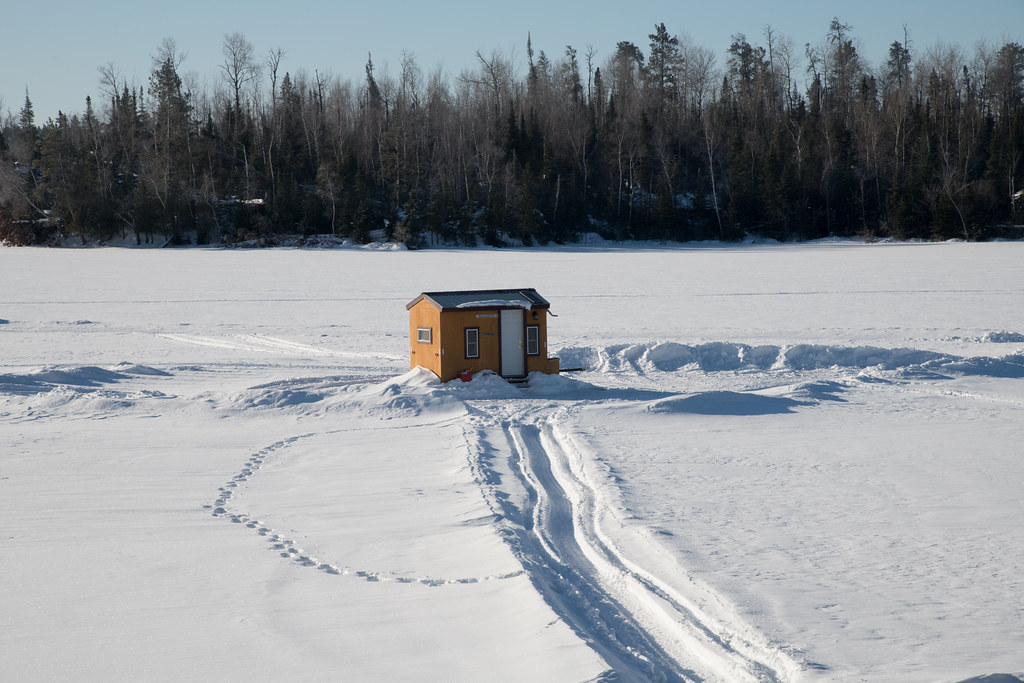In this serene winter landscape, snow blankets the ground, with numerous trails etched into its surface. Dominating the scene is a small, light brown shed positioned at the junction of snow-cleared paths that form a distinct T shape. The shed, featuring a single window and a white door under a slightly pointed gray roof, sits amid a field of snow with a visibly cleared area around it, possibly for ice fishing. Parallel grooves in the snow, likely made by a sled or vehicle, lead to the shed, while distinct animal footprints weave between the paths, adding intrigue to the otherwise quiet scene. Behind the shed, dense rows of tall, wintry trees stretch across the background, their bare branches interspersed with green from evergreen trees, all set against a clear, light blue-grey sky on this bright, beautiful day.